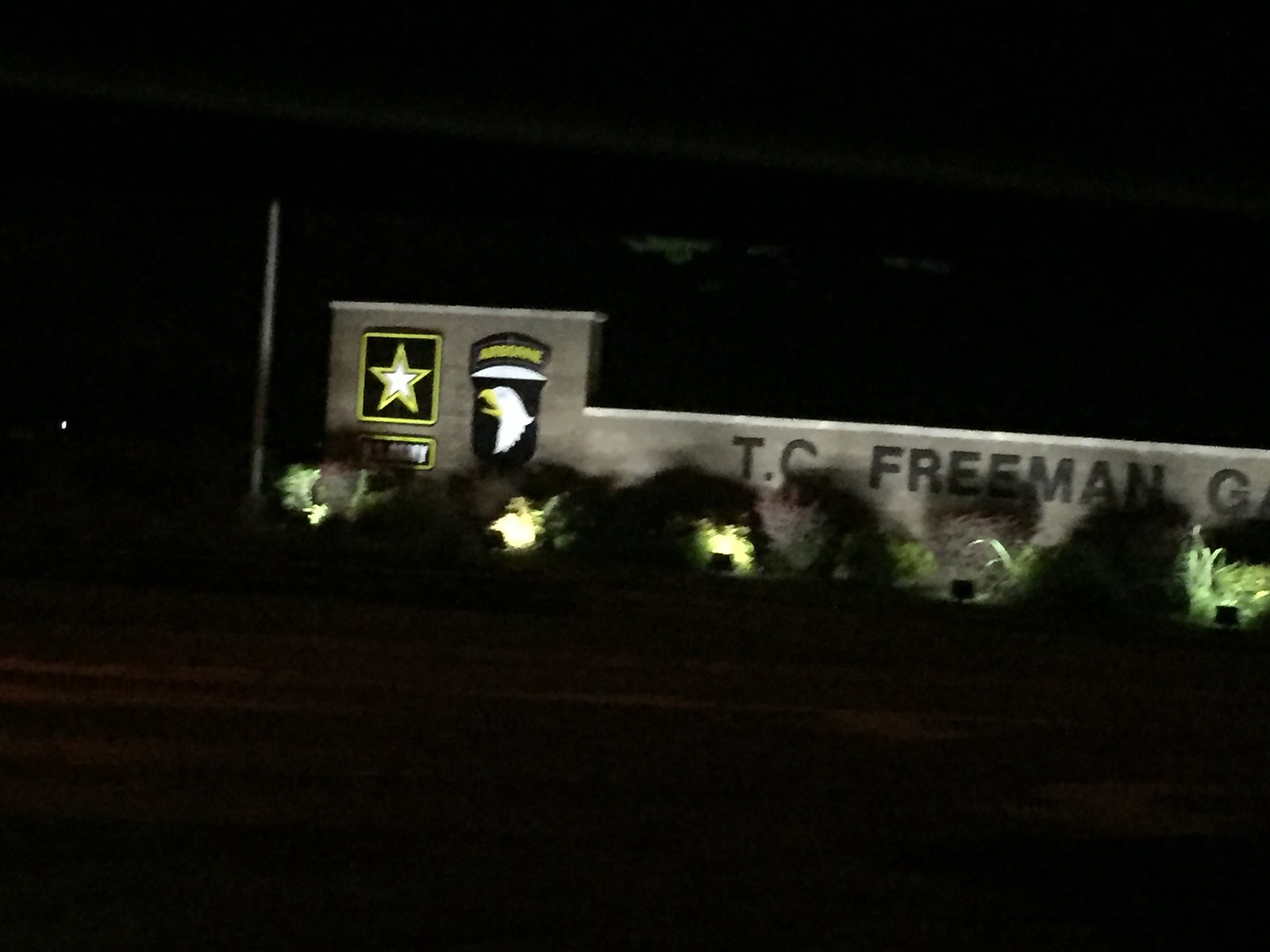This is a nighttime photograph of a U.S. Army training center entrance, featuring a prominent stone structure with gray and lighter-colored stone elements. The structure is illuminated by ground lights and surrounded by green bushes. On the left side of the structure, which is taller and rectangular, there's a black square plaque with a white star and gold border, and below it, another plaque that reads "U.S. Army" in white letters. Adjacent to these is the Airborne badge, depicting a bald eagle with a white head and yellow beak on a black shield with a yellow border. To the right, a long horizontal stone section protrudes, bearing the inscription "T.C. Freeman G" in black letters. The entire scene is set against a dark sky, with a brown telephone pole evident on the left side.